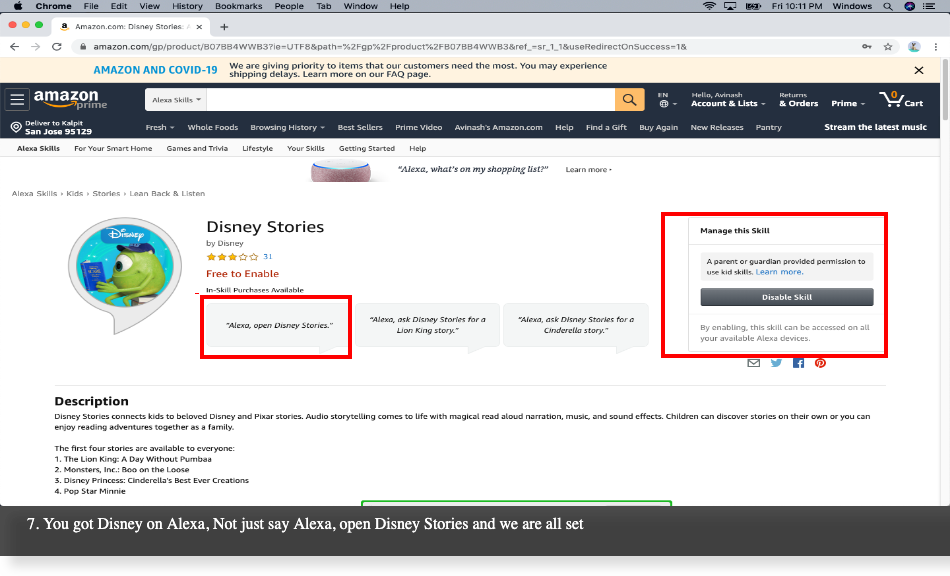A screen capture of an Amazon webpage is displayed on an Apple computer. The image prominently features content related to Disney stories. The webpage appears to be some kind of tutorial, highlighting three key areas with bordered sections that guide the viewer on navigation and button usage. At the top of the webpage, there is a banner discussing Amazon and COVID-19, indicating that this capture is from that pandemic period. At the bottom, a highlighted message provides instructions for accessing Disney stories via Alexa, stating: "To get Disney on Alexa, just say 'Alexa, open Disney stories' and you are all set." This message likely comes from the individual who outlined the buttons, offering helpful tips to the viewer.